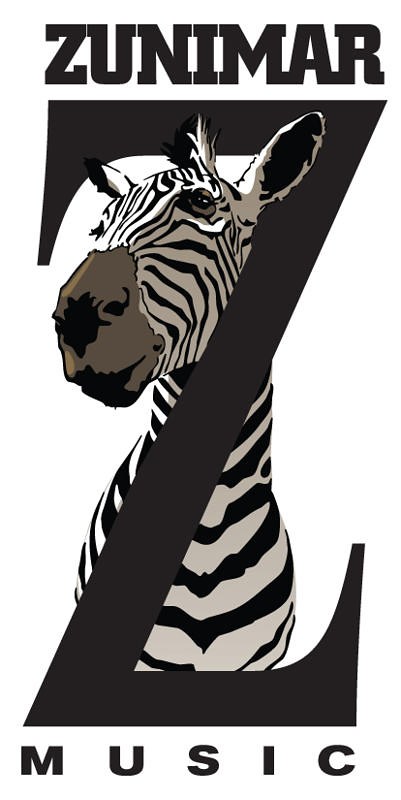The photograph depicts the logo of a company named "Zunimar Music" set against a white background. The main focus of the logo is a stylized cartoon image of a zebra's head and chest, drawn in black and white with subtle gray shading on its muzzle, giving the impression that the zebra is smiling. The zebra is positioned within a large, prominent letter "Z" that encircles its neck and chest. Above this image, the company name "Zunimar" is printed in bold black letters, and below, the word "Music" is similarly displayed in black letters, each character spaced out for emphasis. The zebra appears to be gazing to the left side of the image, and its minimalist yet striking design gives it a distinctive, professional appearance. The logo's color scheme consists only of black, white, and touches of gray, enhancing its bold and clean visual appeal.